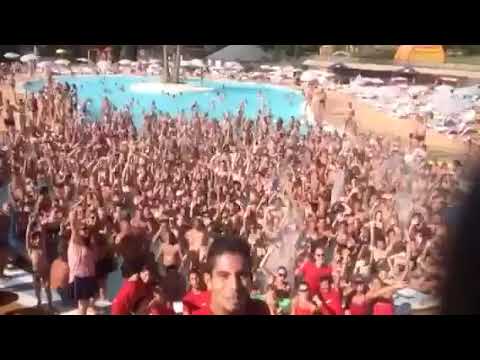This is a full-color photograph of a bustling pool area taken from an elevated point on a bright sunny day, presumably at a water park. Despite the slight blur and out-of-focus quality, the image captures a large crowd of people in swimsuits, most of whom are raising their hands as if cheerfully posing for the camera. The pool, situated centrally in the photograph, is filled with vibrant blue water, and some people appear to be enjoying it. Notably, at the top and bottom of the image, there are horizontal black strips framing the scene.

The pool area is surrounded by numerous attendees, suggesting a summer celebration or vacation. Near the camera, a group of people wearing red t-shirts, possibly park staff, can be seen, with one individual, a man with dark hair and a goatee in a red top, standing out more prominently in the foreground. Surrounding the pool are chairs intended for sunbathing and beach umbrellas, providing shade. Additionally, in the upper left corner, several beach umbrellas are visible, and in the upper right corner, there is a yellowish structure. In the center of the pool, a small island with what appear to be coconut tree stumps adds visual interest to the scene.